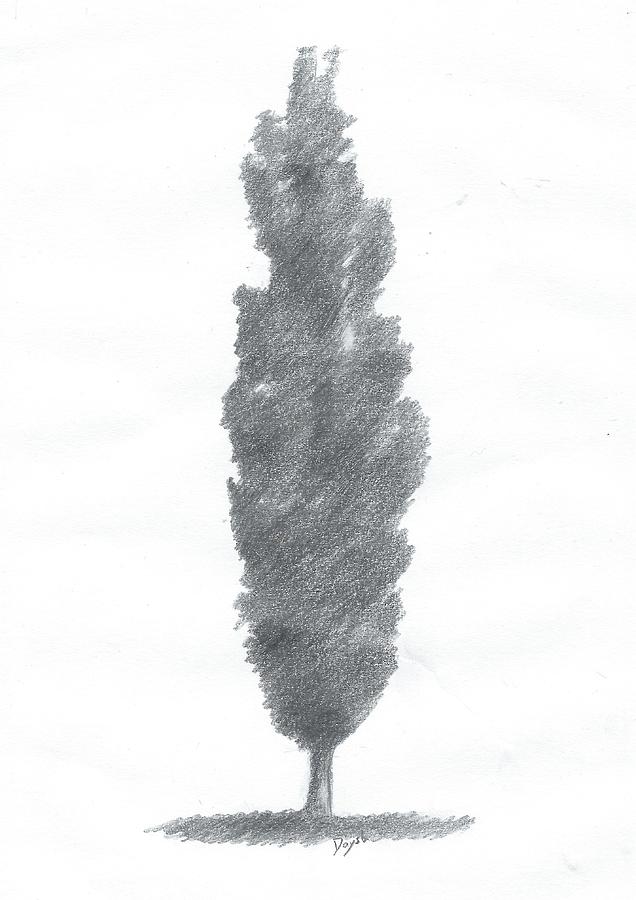This image is a detailed charcoal pencil drawing on a white paper background, characterized by its black and white color scheme and lack of sharp details. The artwork depicts a tall, narrow tree standing in a small patch of grass. The tree, which resembles a spruce, has softly drawn foliage without distinct branches, giving it a smooth, almost silhouette-like appearance. The background of the image is predominantly pure white, showing subtle textures that hint at the paper material. Beneath the tree and grass, there is a small circle containing the artist’s initials, which appear to spell "Y-A-Y-S-A" or "D-O-Y-S," though the exact letters are somewhat unclear. The overall form is sketchy yet dense, with broad strokes that convey the essential shape and texture of the tree, leaving viewers with a clear understanding of the scene despite the lack of fine details.